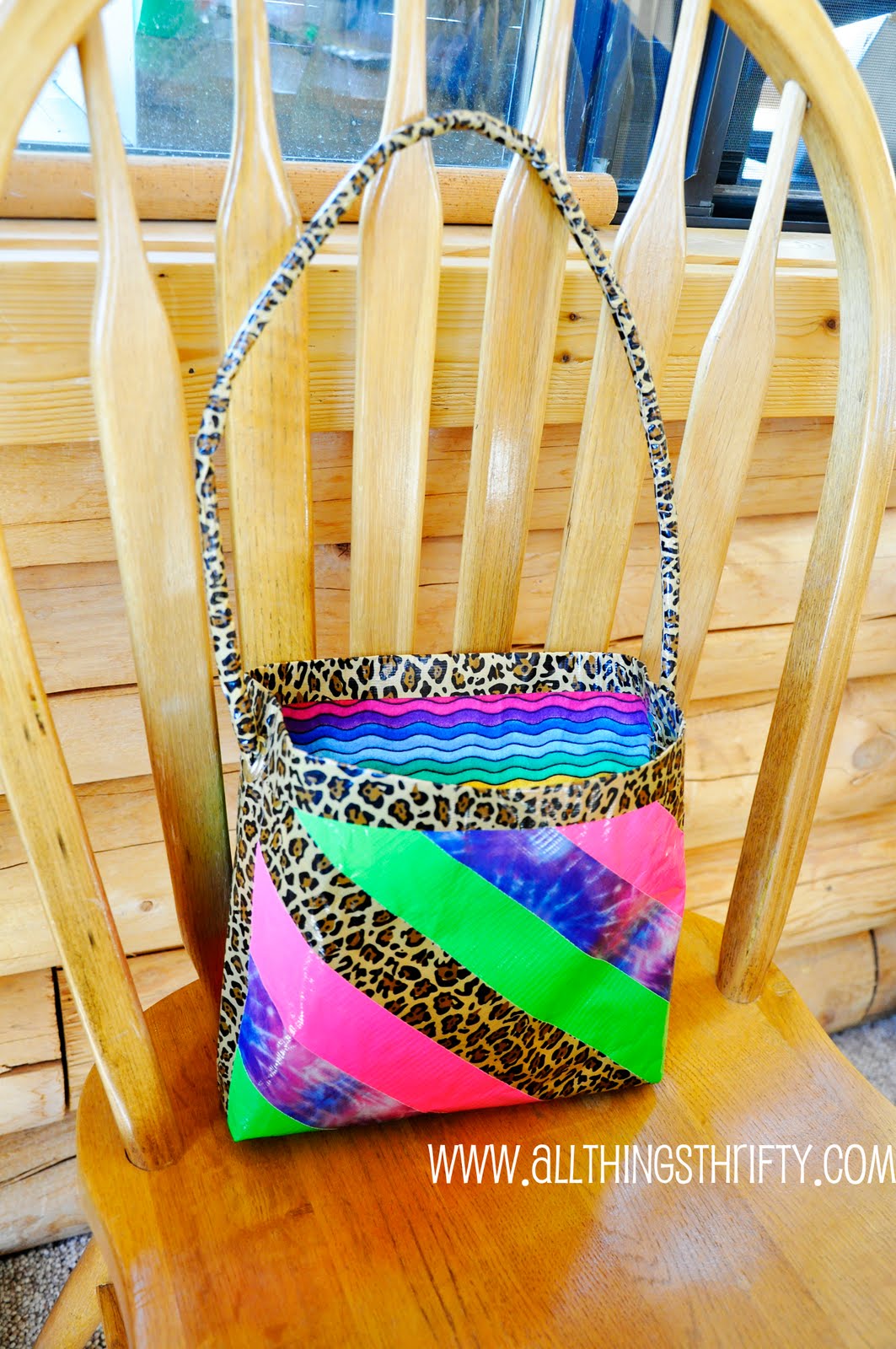In the image, a vividly colorful handmade purse is prominently displayed on a light-colored wooden chair with a glossy lacquered finish. The chair is positioned against a matching wooden wall, which includes a window and what appears to be a wooden dowel or rolling pin on the windowsill. The purse itself is a striking ensemble of various vibrant fabrics, featuring blue batik-like waves, neon green, hot pink, purple gradients, and rainbow patterns. The purse is edged with a distinctive leopard skin print that also forms its handle. Adding to the eclectic look, the photo includes text at the bottom, in white capital letters, reading "www.allthingsthrifty.com," with the only lowercase letter being the 'a' in 'all.' The background of cohesive wooden elements contrasts sharply with the purse's chaotic burst of colors and prints.